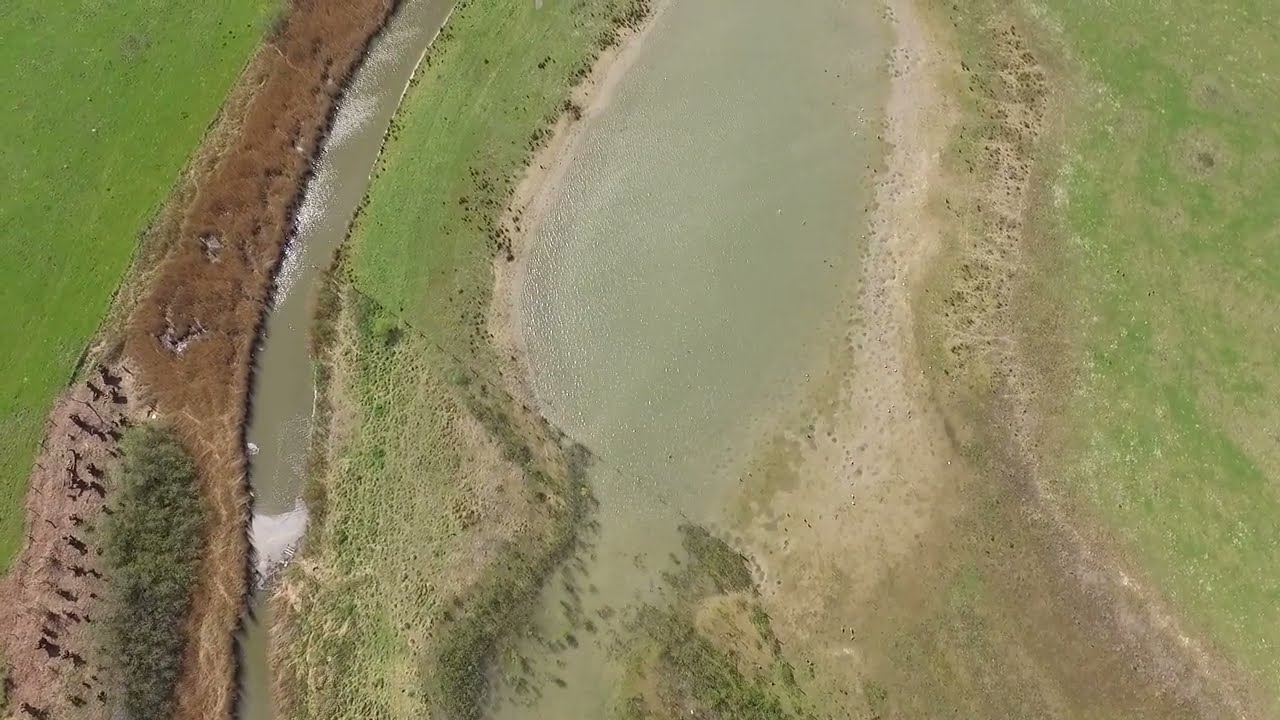The image captures a bird's eye view of a diverse and vibrant landscape. At an elevated vantage point, the scene features a notable river flowing from the bottom edge to the top edge along the left side of the image. The river's water has a distinct brownish tan color, and a small section of rapids can be observed near the bottom. To the left of the river, there's a brown bank transitioning into a lush expanse of grassland.

Moving further left, the top left-hand corner of the image showcases the greenest and most lush area. Adjacent to this verdant section is a strip of predominantly brown terrain, with sparse patches of green, suggesting dried vegetation or a sandy expanse.

To the right of the river, the landscape continues with another grassy bank leading to a pond, which features a water color distinctively milky gray. The area surrounding the pond also displays patches of sand and less vibrant green foliage.

Towards the center right of the image, another significant body of water, potentially another pond, can be seen. It exhibits a lighter shade of the same olive green color as the previous body of water. Alongside it, there is a sandy strip interspersed with some vegetative growth.

The right-hand side of the image concludes with a deep green area, not as lush as the greenery on the far left, fading into a field or potentially a sectioned-off farming area. The spatial arrangement emphasizes the juxtaposition of different natural features, including varied water bodies, vegetation, and soil types, presenting a rich and detailed panorama.